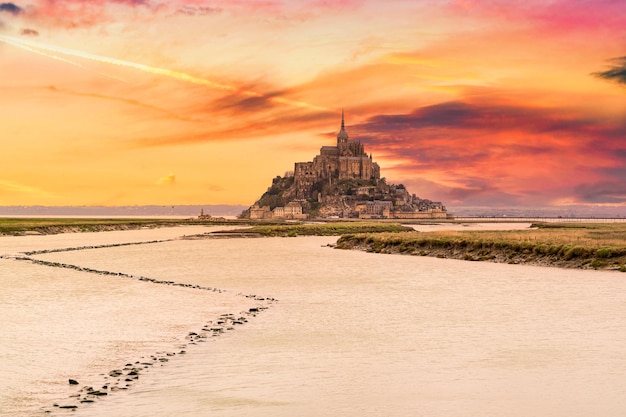The photograph captures the breathtaking scenery of Mont Saint-Michel at the edge of a beach during what appears to be either sunrise or sunset, as indicated by the vivid hues of yellows, reds, oranges, and pinks that bathe the sky. Dominating the background is the iconic medieval-style castle perched atop the mount, which is surrounded by a compact town. The fortress-like structure, built right at the edge of the water, seems to majestically rise from a rocky, hill-like foundation. In the foreground, a sandy beach stretches out, interspersed with grassy patches and ditches. A narrow path made of rocks winds its way from the beach up towards the distant castle. The picturesque scene is further enhanced by a single ray of light piercing through the rich, colorful sky to touch the tallest spire of the castle, adding a mystical touch to the already enchanting view.